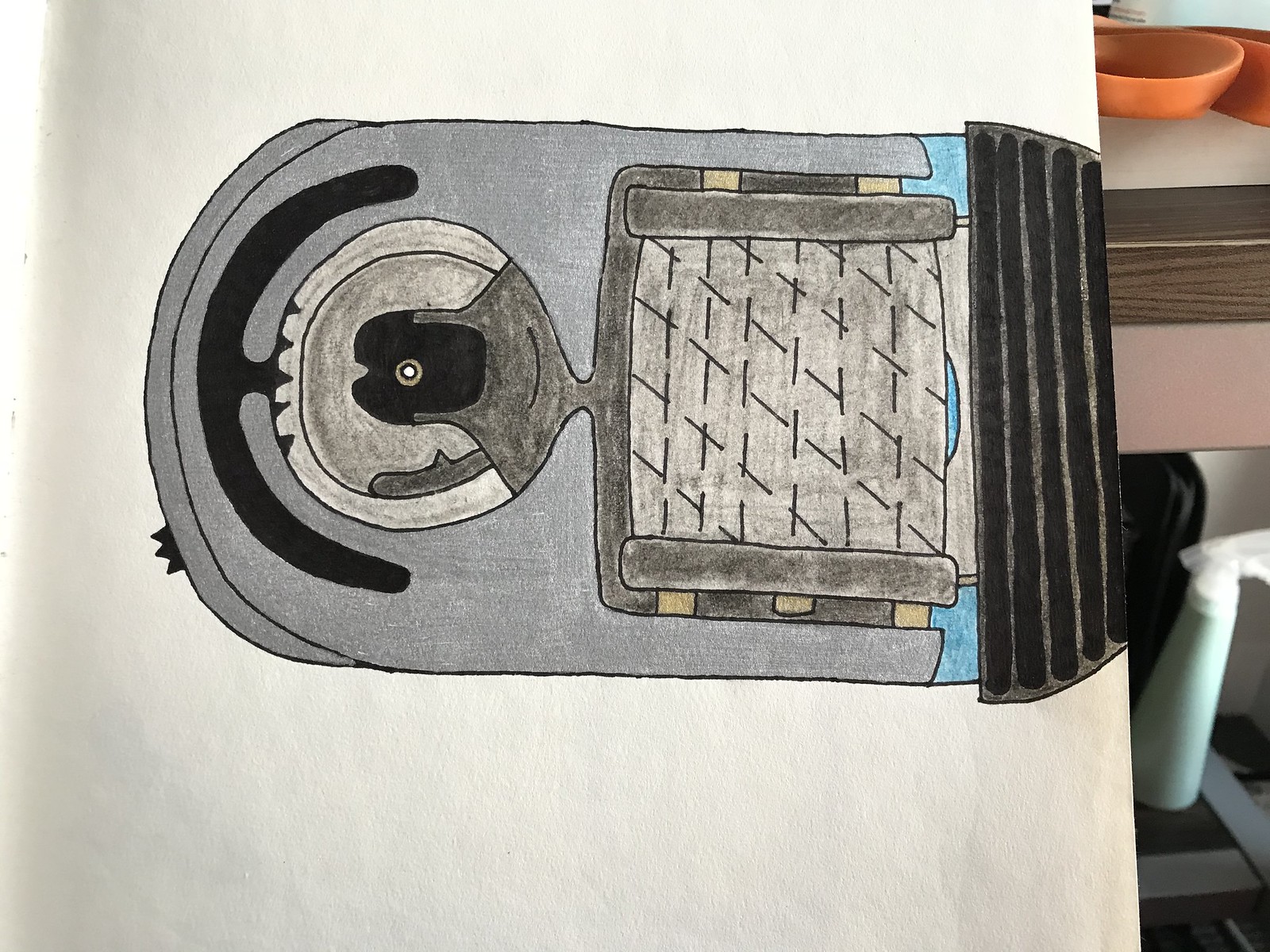The image features a detailed sketch drawn on a piece of white paper, oriented sideways. The sketch depicts a vintage, arch-shaped radio, predominantly shaded in gray. The artist has meticulously included a circular tuning dial on the front of the radio, as well as an arched design accent shaded in black and gray. The speaker area is illustrated with a grid pattern, featuring horizontal lines intersected by vertical ones. The medium used for the artwork appears to be either colored pencil or marker, providing a bold and defined look. The photograph capturing this sketch was likely taken in a kitchen setting, as evidenced by the presence of orange bowls and other assorted items on a shelf in the background.